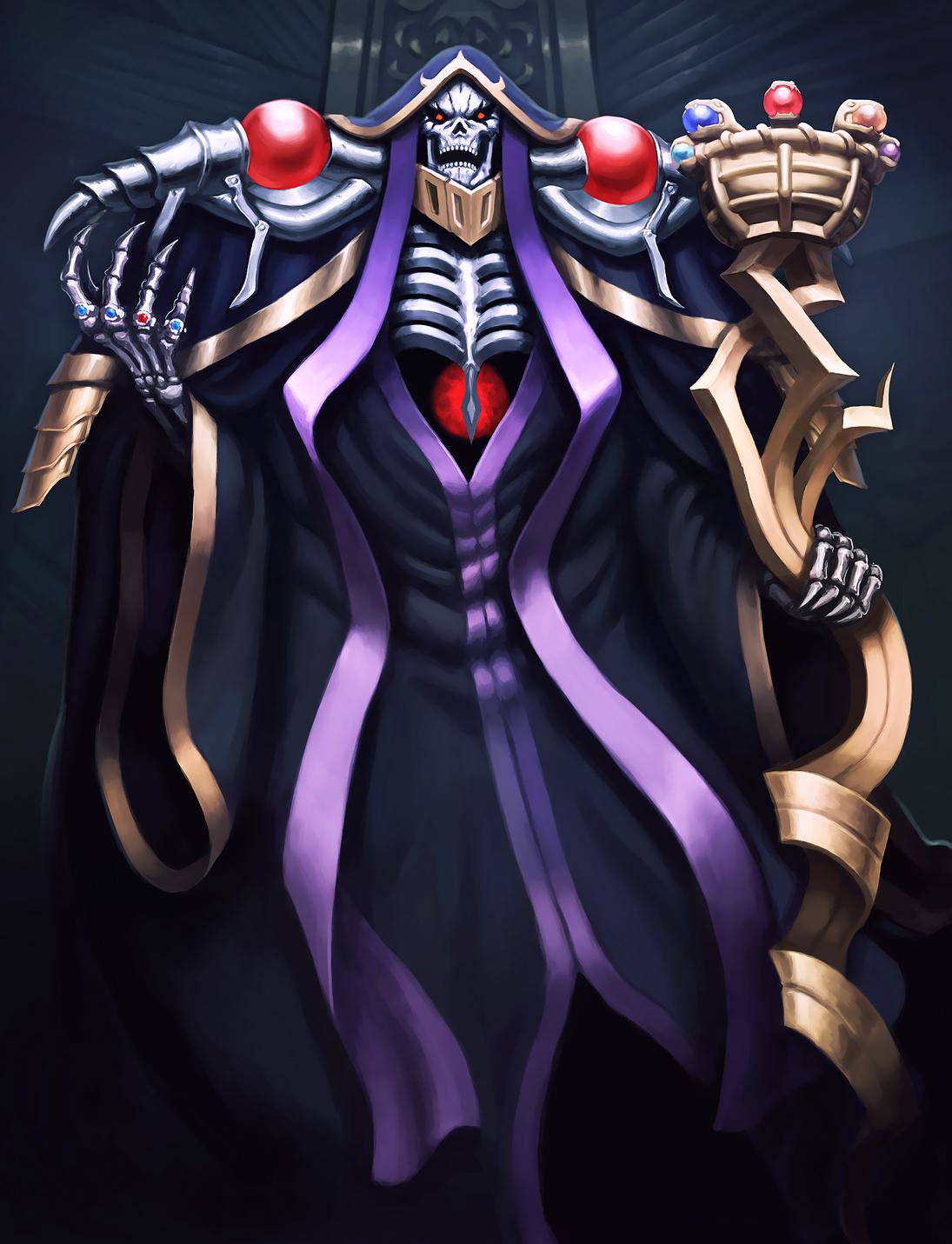The image is a detailed, computer-generated graphic of a menacing skeleton character reminiscent of Skeletor. The focal point is a cartoony skeletal face with red, beady, glowing eyes, roaring in fury. His attire is a black robe adorned with purple piping and fringes, complete with a helmet featuring a gold edge and a blue top. Notably, there are metallic silver arms with red, bulbous shoulder pads emerging from his robe, adding to his intimidating presence.

The skeletal figure holds a golden staff, adorned with a series of colorful gems—light blue, dark blue, red, orange, and purple. His skeletal hand is also decorated with rings in various shades of blue and a single red gemstone. He possesses a gold jaw protector, and below his exposed ribcage, a glowing red orb suggests a heart-like element.

Behind him, a massive, ornate throne serves as the backdrop, featuring gold metallic swirls and additional decorative elements. On the right side, there's a golden cup embellished with colorful jewels and topped with gold snake heads, holding orbs in blue, red, and gold, with a twisted golden handle that the skeleton grips. The entire scene is set against a stark black background, enhancing the eerie and striking visual impact of the character.